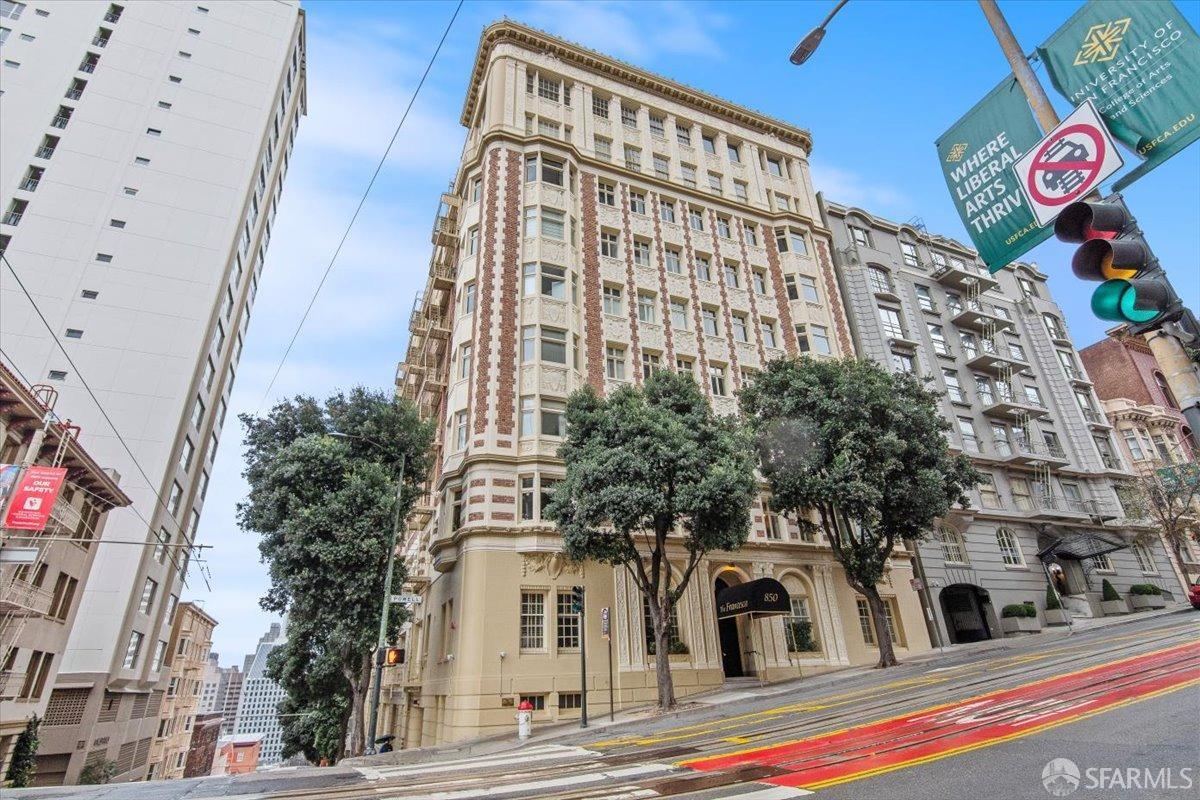The photograph captures an urban scene likely in San Francisco, characterized by its distinctive sloping streets and cable car tracks. The image showcases a blend of architectural styles with several taller buildings predominantly in tan and gray hues. The foremost structure is a light tan-colored Art Deco building with brown designs, estimated to be around 10-15 stories high. Adjacent to it stands a slightly smaller, gray building. Both buildings are set against a backdrop of more city structures visible as the street descends. 

In front of these buildings, there are a few trees breaking the monotony of the concrete landscape consisting of roads, sidewalks, and trolley tracks. The street itself has a distinctive appearance with red and yellow lines running along its gray surface. On the far left, partially visible, is another tall apartment building that adds to the city's dense architectural tapestry.

The right side of the photograph features a traffic light mounted on a pole adorned with green banners. One banner states “Where Liberal Arts Thrive” and the other indicates “University of San Francisco,” hinting at the educational presence in the area. Additionally, there's a sign with a red circle and a line through it, likely indicating a railway crossing. The ambient overcast sky with blue patches provides a subdued backdrop to this vibrant urban landscape.